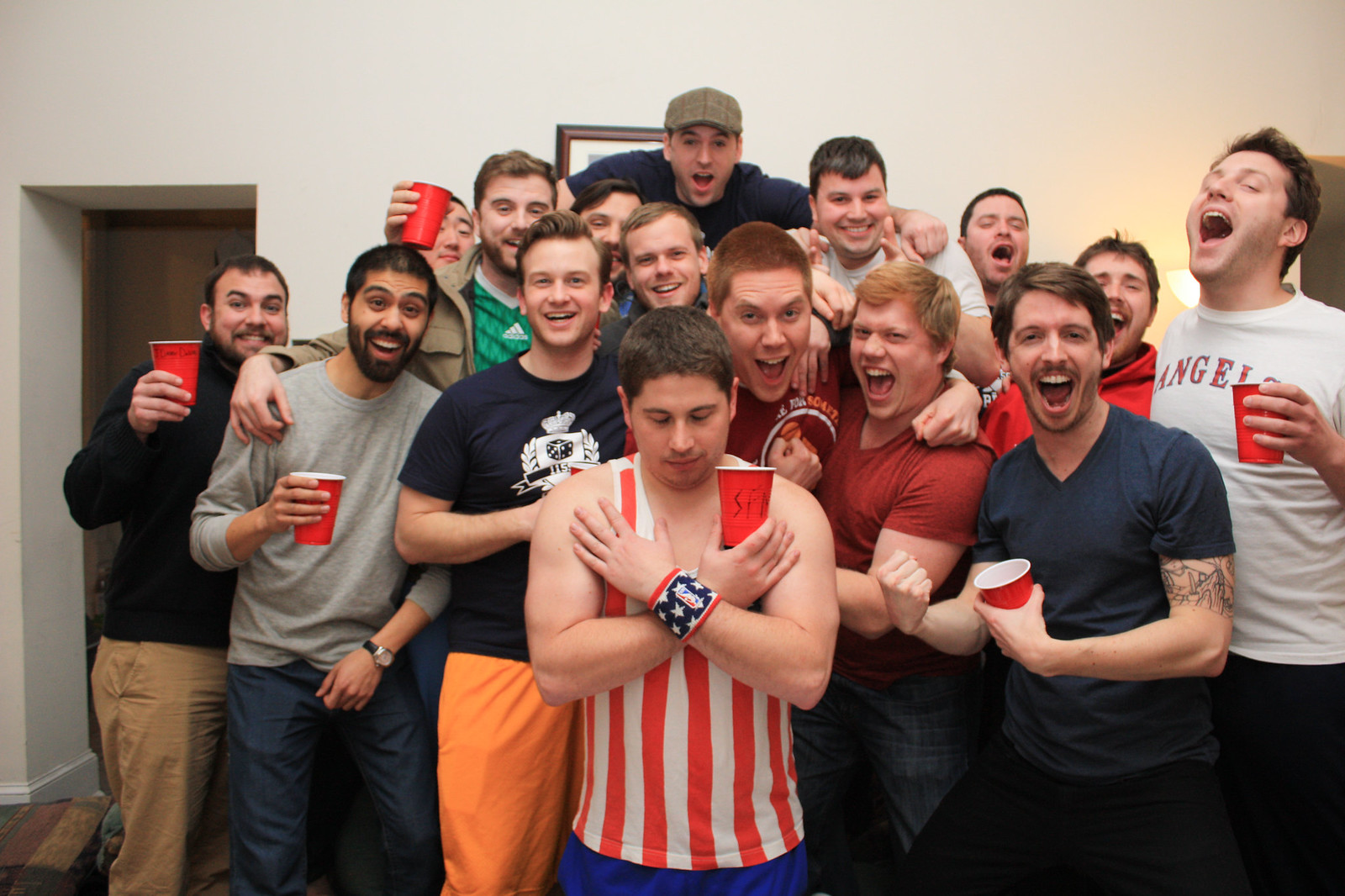The photograph captures a group of approximately 15 men, likely fraternity brothers, who appear to be in their late teens or early twenties, posing together in an interior setting with a white-painted wall and a brown wooden door frame to the left. The floor is made of wooden planks, and a partially obscured brown picture frame hangs behind the group. The majority of the men are Caucasian, though there is a man with darker skin wearing a gray long-sleeved shirt and blue pants, possibly Hispanic, and an Asian man peeking out from behind a red solo cup. Most of the men are holding red and white plastic solo cups, suggesting a party atmosphere. The man on the far left, in a black long-sleeved shirt with khaki pants, raises his cup in the air. The men are mostly wearing casual t-shirts and appear to be mid-yell, adding to the playful and rowdy vibe. In the center, a man stands out with his arms crossed over his chest and his head bowed, eyes closed, as if being humorously reverent. The scene is lively, with the men closely grouped, creating a sense of camaraderie and festivity typical of a fraternity gathering.